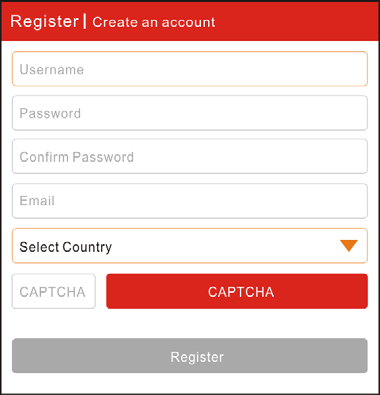The image depicts a registration form positioned inside a square frame with a dark gray border. At the top of the form is a horizontally stretched red box spanning from the left edge to the right edge, containing the text "Register/Create an Account". Below this title are several input fields outlined in a light orangey-red color.

The first field is labeled "Username". Following this is the "Password" field, and immediately below it is a "Confirm Password" field. Next, there is an "Email" input box. Beneath the email field lies the "Select Country" dropdown box, which is currently highlighted and features a downward arrow in an orangey-red hue. 

The left side of the form includes a CAPTCHA section, bordered in gray, with a longer orange box stating "CAPTCHA" in white. 

At the bottom of the form, there is a gray "Register" button. The entire layout is neatly encased within the dark gray border, which encloses the rectangular form, giving it a structured and defined appearance.